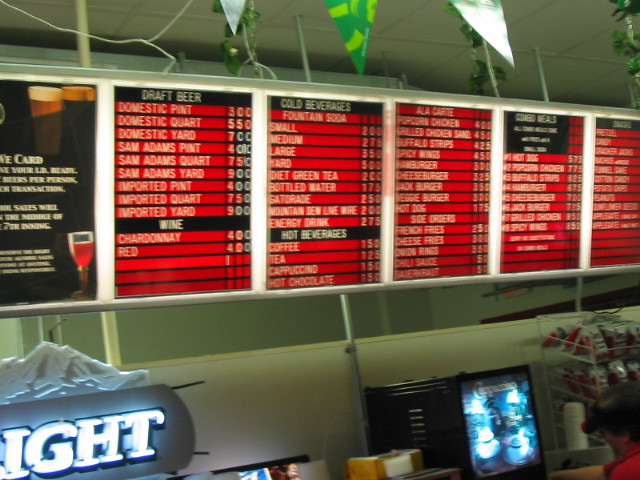In this detailed photograph taken inside a restaurant, the focus is on the overhead menu display. The menu descends from the ceiling about an inch before angling to the right, providing a clear view of the various food and drink options. The ceiling itself is white with a rectangular drop design, segmented by white borders. 

In the left corner of the image, a white wire descends, curves inward about two inches, and then veers off to the right. Another similar wire trails down, angles right, and disappears behind the sign. In the background, about two inches behind the sign, you can see a white pole, followed by another one six inches farther in, and another pole about two inches from the right side of the image, supporting the sign from the ceiling.

At the top of the image, there is a glimpse of a silver flag with a hint of greenery, accompanied by a green and yellow flag to its immediate right, and another silver flag with greenery beyond it. Additional greenery is visible in the far right corner. 

The menu is partially obscured, but you can identify two drinks in the top right corner, with a red drink in the bottom corner. Each menu section is demarcated by white borders. The first visible section lists draft beers in black bordered text, followed by the detailed beverage list. Beneath it, a section details the wines available. 

The third section, marked by a black border, displays 'Cold Beverages' with an accompanying list, followed by another section for hot beverages. The subsequent section lists sides like French fries and hot dogs, about 12 items in total. To the right is a 'Combo Meals' section in black border; however, some of the lettering is not visible. The remaining items extend off-screen.

Below the menu is a white wall. To the left, a partial Coors Light sign is visible, displaying only 'IGHT'. The sign is silver, with white illumination. Slightly off-center to the right, a black cappuccino machine with blue accents faces right. In front of the machine, at the bottom right corner of the image, stands a person wearing a red shirt, glasses, and a visor.